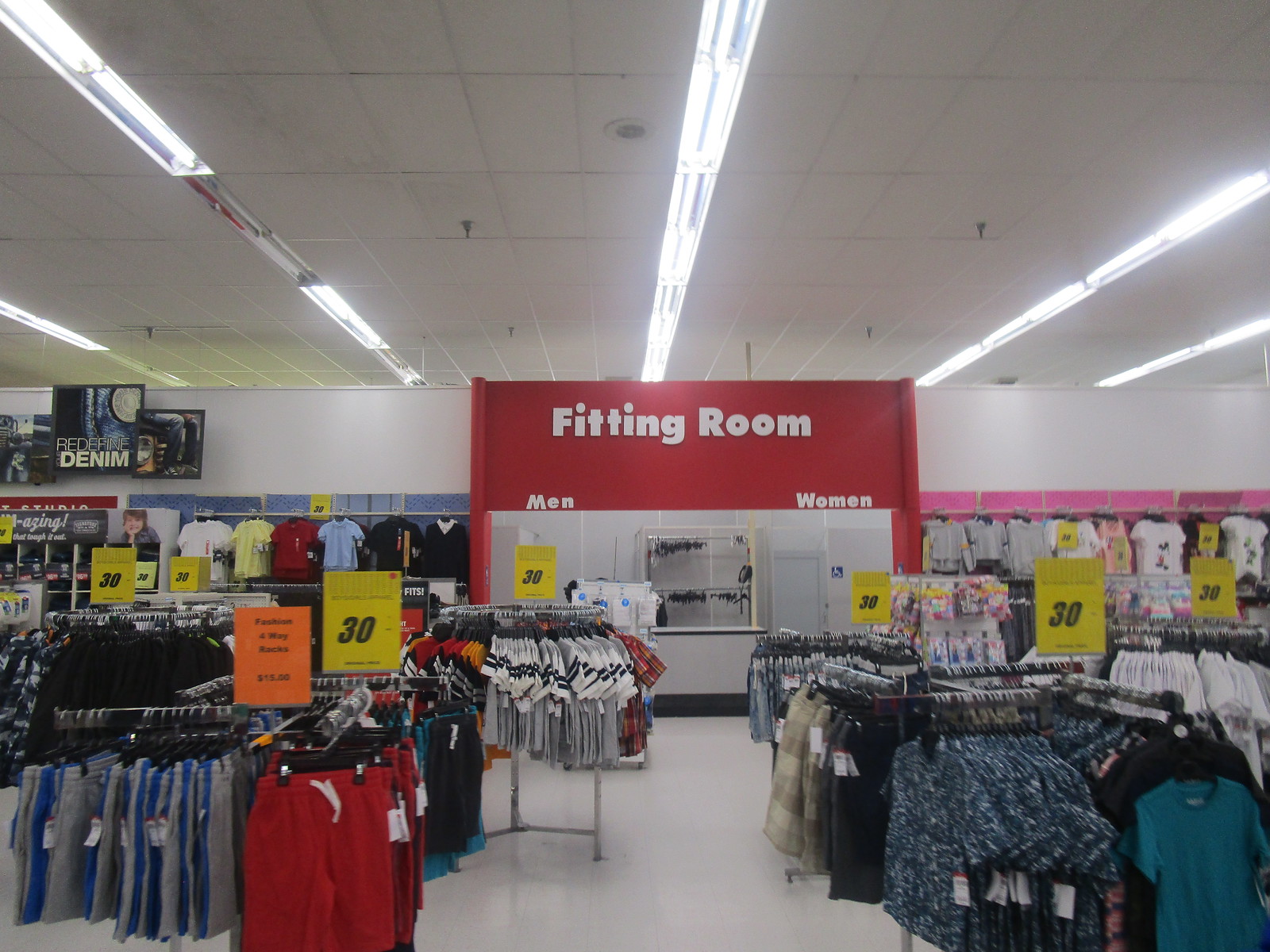This photograph captures the vibrant clothing section of a retail store. In the foreground, several black clothing racks display an eclectic assortment of apparel in a wide array of colors, including teal, navy with white patterns, red shorts, and gray and blue shorts. The background features more colorful t-shirts neatly arranged. Atop the clothing racks, numerous yellow signs with black font prominently advertise a 30% discount. The image also reveals a red wall in the background, adorned with white text indicating the fitting rooms for "Men" and "Women," separated into two distinct sides. Overhead, the white drop ceiling houses fluorescent lighting fixtures and visible fire sprinklers, contributing to the store’s functional ambiance.